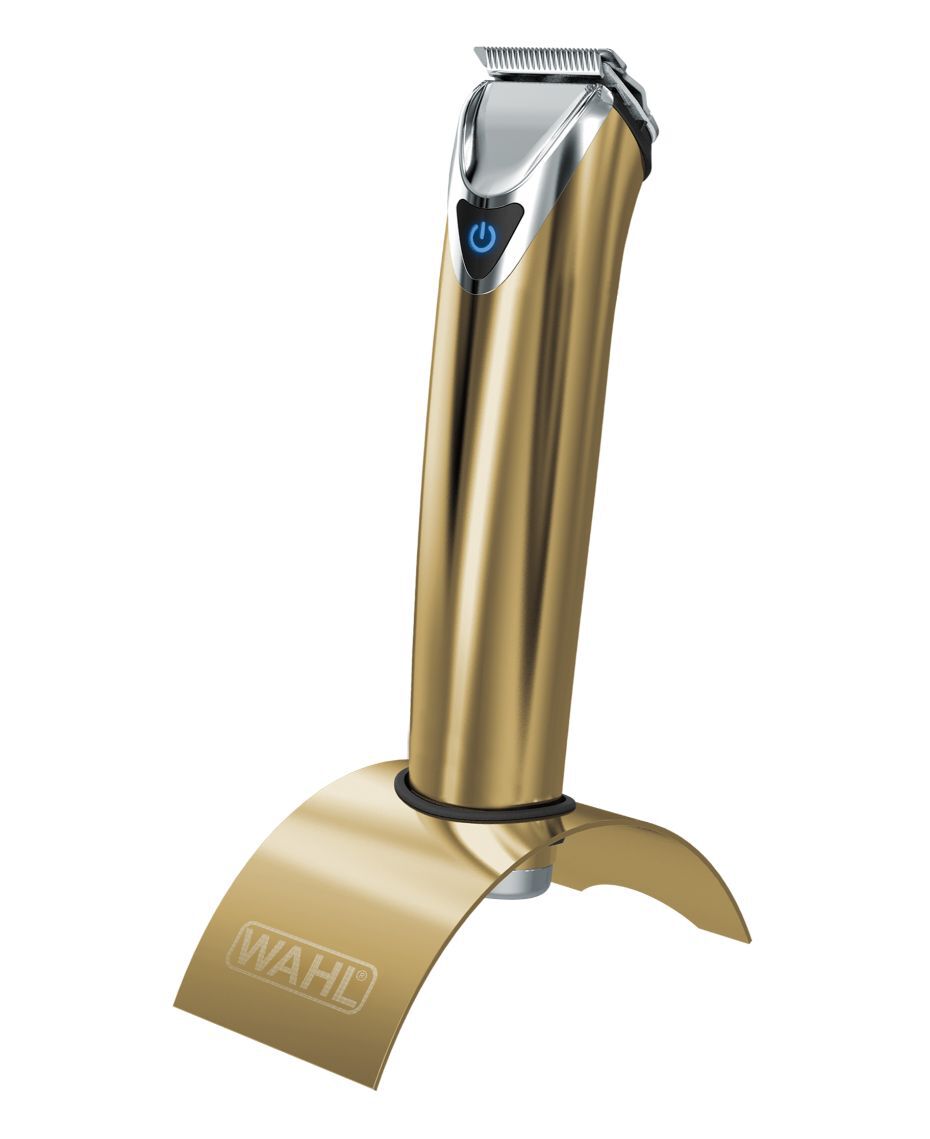This image showcases a luxurious pair of electric clippers prominently featuring a shiny golden body, especially striking at the cylindrical base and curving upward to the bladed top. The top section, housing the blades, transitions to a silver tone and forms a stylized rounded triangle. A black power button is positioned within this silver section, featuring a blue light on the button itself, marked by a circle interrupted by a blue vertical line. The blades appear to be silver in color. The clippers are branded with the label "WAHL," etched on the base. They are presented on a unique metallic stand—also branded with "WAHL"—shaped like a half-circle with a central indentation that securely holds the clippers. The stark white background emphasizes the clippers and stand, ensuring no distractions from the product’s sleek and modern design.